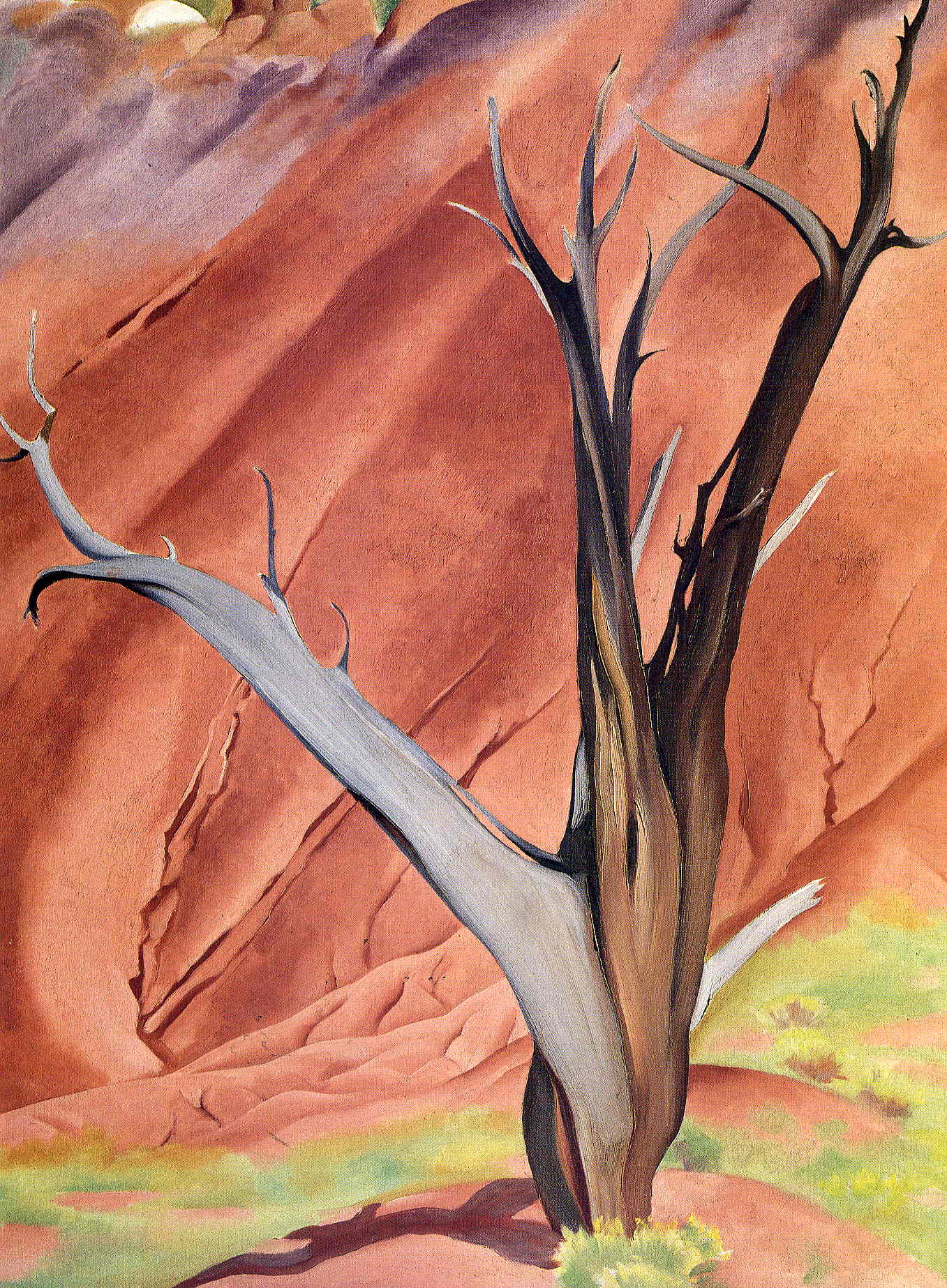"Gerald's Tree" by Georgia O'Keeffe is a vertical rectangular painting in the American modernism style, characterized by its surrealistic and southwestern art influences. The painting centers on a seemingly dead, petrified tree trunk that stands prominently from the bottom center to the top of the composition. This tree splits into three primary branches: one on the left, a grayish hue curving slightly at its tips; the central branch, a blend of dark and medium brown, rising straight up with minor curves at the ends; and the right branch, mostly dark brown, extending towards the upper right corner.

The backdrop of the image vividly portrays a southwestern landscape. The foreground consists of reddish-pink, small rolling hills interspersed with patches of green and yellow grass and flowers. The middle to the upper part of the painting transitions into a rugged, mountainous cliffside, with visible cracks illustrating the raw texture of the rock. This reddish-pink cliff gradually fades into a purplish hue at the top, enhancing the surreal, dreamlike quality of the scene. The overall color palette is composed of earthy tones including shades of green, yellow, burnt orange, and muted purples, reflecting the natural southwestern terrain.